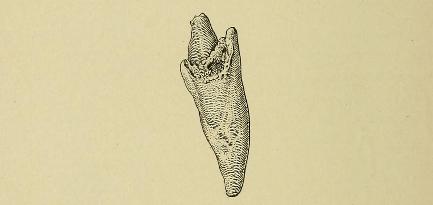This image features a highly detailed pencil or black ink drawing centered on a beige or light brown rectangular sheet of paper, possibly construction paper. The drawing itself is rendered in black and showcases an elongated, slender, triangular object. The base and background are a muted brown color, lending a neutral palette to the whole piece. The drawn object features a pointy bottom that gradually broadens before tapering back to a dull top, resembling a tooth, claw, or perhaps a plant bud or root. Textural details are emphasized through horizontal and vertical lines, adding depth and dimension. The overall appearance is slightly ambiguous, with some suggesting it resembles a fossil, a horn, or a nail. The intricate linear patterns suggest various textures woven into the structure of the object, enhancing its complexity and visual interest.